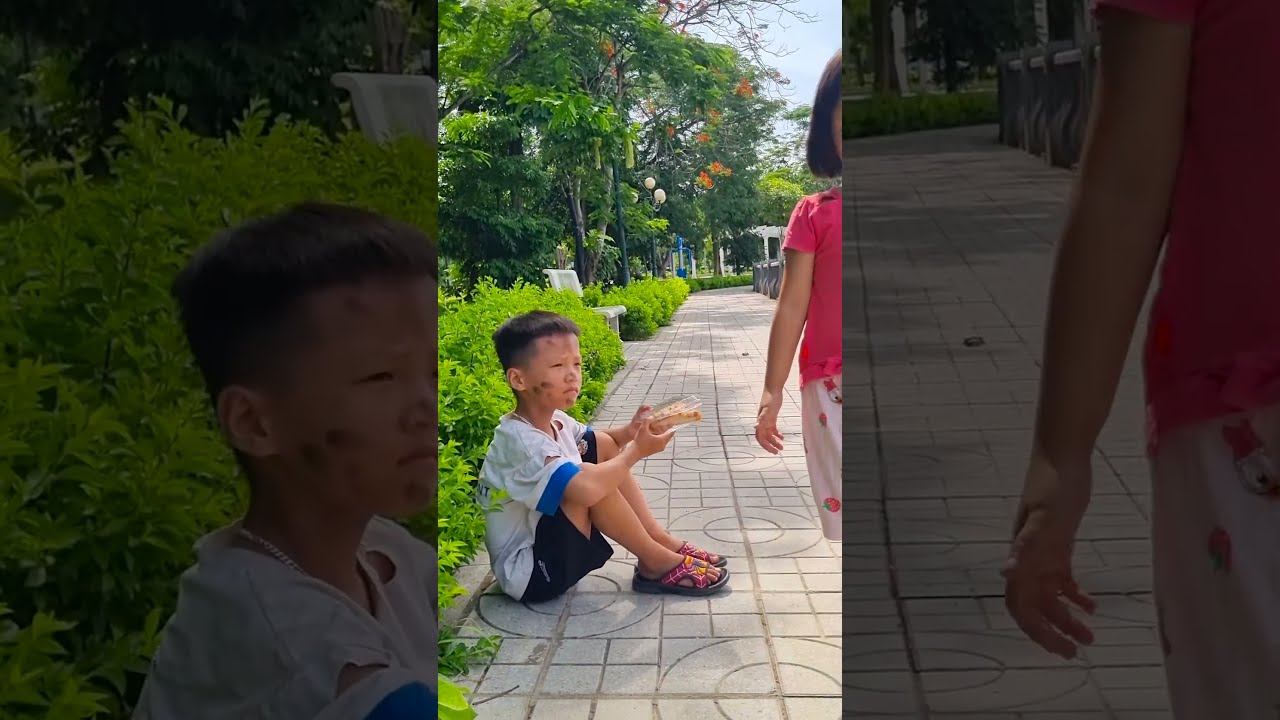The photo is a composite image with a portrait-oriented photograph layered over an enlarged, darker-toned landscape version of itself. In the center of the image, a young boy, around four or five years old and of Asian descent, sits on a patterned concrete sidewalk. The sidewalk features embedded circular patterns and is bordered by lush, green landscaping, including a garden with colorful trees and hedges. The boy has short black or brown hair in a fade haircut and a dirty face marked by what appears to be black fingerprints. He wears a loose-fitting white t-shirt, dark shorts, and Spiderman-themed sandals. He holds a plastic clamshell container, possibly with food, in his hands, which are folded in front of his knees. The boy's attention is directed toward a young girl walking past him. Only the girl's arm, a portion of her short black hair, her pink shirt, and possibly white shorts with a strawberry or a character design like Daisy Duck are visible. 

The enlarged sections on the left and right of the composite image provide close-ups of the boy's face and the girl's arm, respectively, emphasizing the central elements of the photograph. The entire scene is set against a backdrop of green hedges and a garden, enhancing the vivid color and natural setting of the composition.